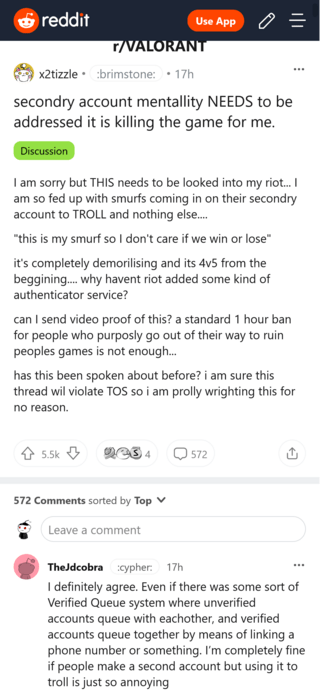The image shows a mobile browser in portrait orientation, displaying the Reddit website. At the top-left corner, the recognizable Reddit logo is visible. To the right, there's a prominent red button labeled "Use App" in white text, and next to it is a small pencil icon for editing alongside lines indicating expandable menu options.

Below this header, the subreddit "r/Valorant" is clearly identified, followed by a user post stating: "Secondary account mentality needs to be addressed. It is killing the game for me." Accompanying the post title is a lime green tag marked with "Discussion" in black text.

The post continues with the user elaborating on their concerns and opinions about the issue at hand. Following the content, interactive elements include an upvote and downvote arrow, the number of current comments, and indicating the presence of one comment below the post.